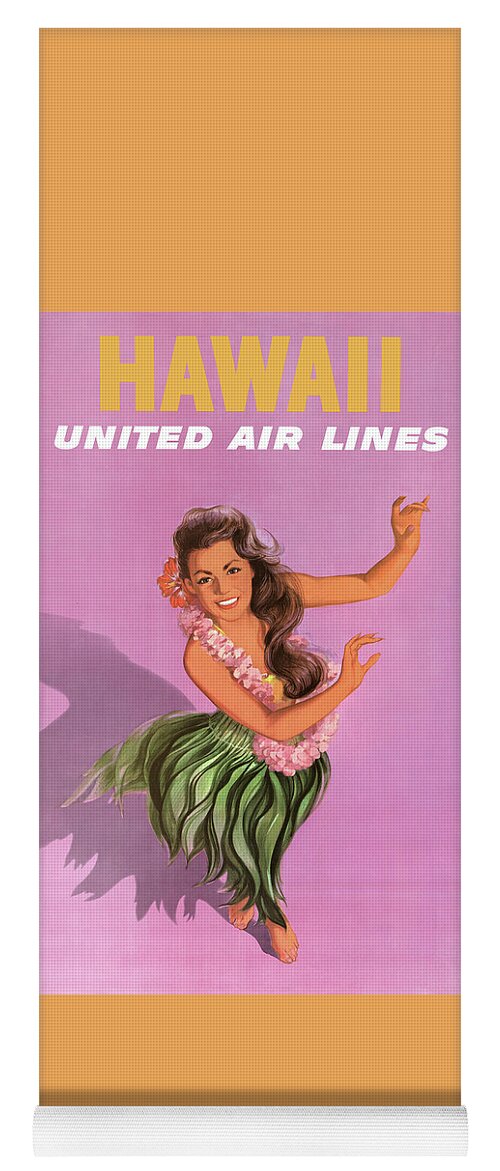This image appears to be a vintage promotional poster for United Airlines, likely from the 1930s or 40s. The poster is vertically rectangular with distinct border elements: a white stripe at the bottom, topped by a dark brown line, and lighter brown borders at both the top and bottom edges. The main background color is a pinkish-purple hue. At the top of the poster, in large, all-capital orange letters, is the word "HAWAII," with "UNITED AIRLINES" written below it in smaller, white, italicized capital letters.

The central illustration features a young woman with long, brown hair and a red hibiscus flower tucked behind her ear. She is depicted in mid-hula dance, her arms gracefully extended. She wears a traditional green grass skirt and a pink flower lei draped around her neck. She is smiling and looking up at the viewer, positioned slightly from an elevated perspective, casting a shadow on the purple-pink background behind her. Her bare feet and hands emphasize her carefree and joyous demeanor, capturing the spirit of classical Hawaiian dance. The overall artistic style and design elements suggest the poster is both a piece of art and an advertisement aimed at enticing viewers with the exotic allure of Hawaii.